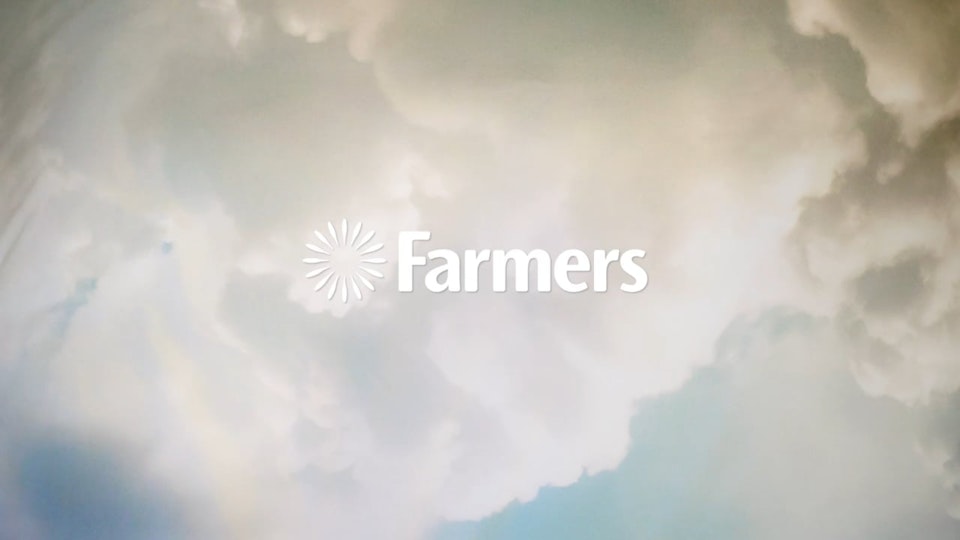The image is a horizontally rectangular advertisement for Farmers Insurance, featuring a serene yet dynamic sky scene. Dominating the background is a photograph of a cloudy sky, with the left two-thirds filled with large, fluffy white clouds, and the right edge showcasing darker, gray clouds that hint at impending rain. Along the bottom edges, patches of clear blue sky peek through. Centered prominently is the word "Farmers" in bold white letters, with a capital F and the remaining letters in lowercase. To the left of the text is a circular white logo resembling a sun, complete with rays or petals extending outward. This cohesive and balanced visual seamlessly integrates the brand name and logo against a picturesque sky backdrop.